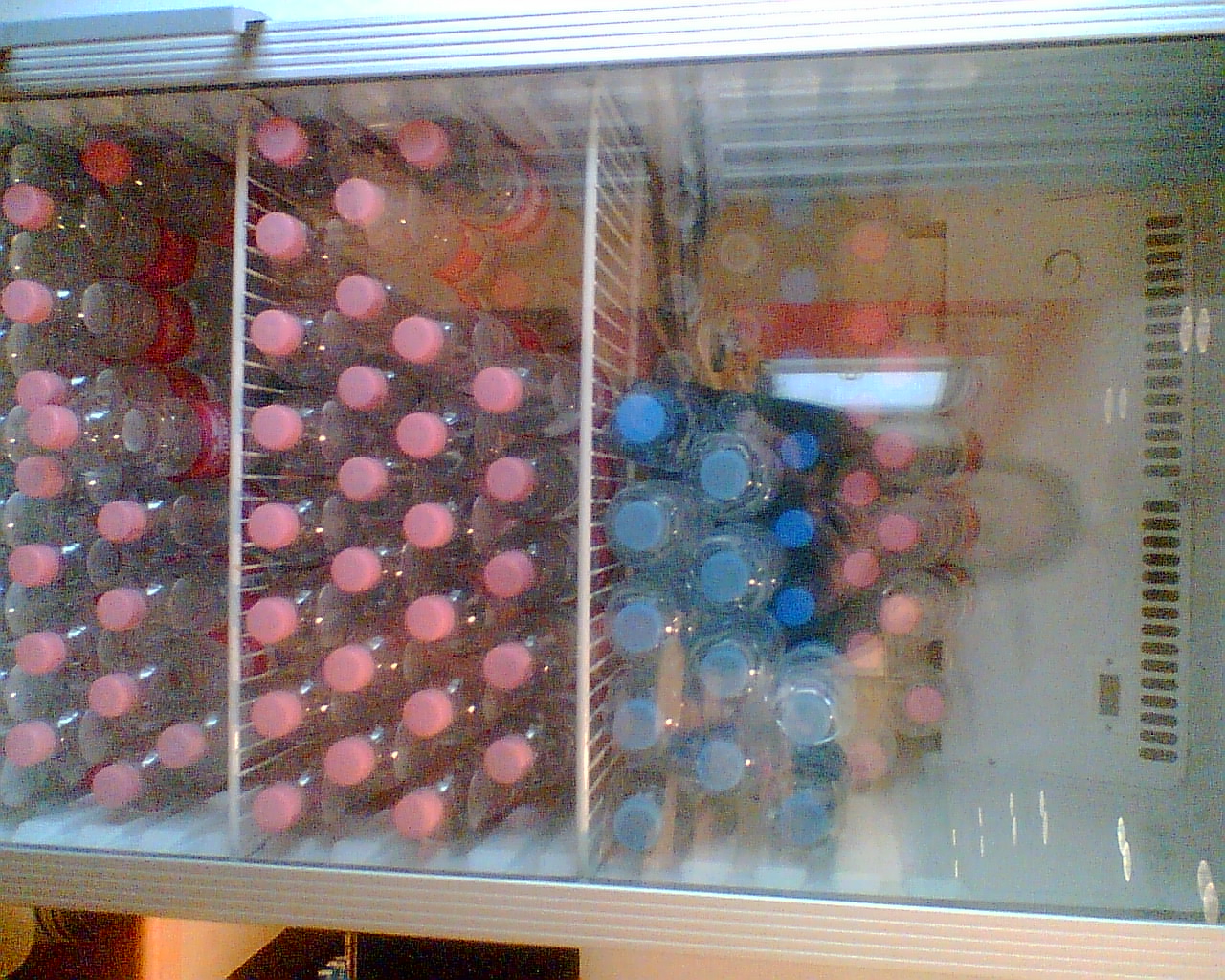This detailed image captures a cooler, likely located in a store, filled with numerous clear plastic bottles, each containing a clear liquid which could be water or another beverage. The cooler is closed, with a glass top through which everything inside is visible. The cooler is divided into three parts by white wire racks. 

The majority of the bottles—about 80%—have pink caps, densely packing the middle and left sections. To the right, there are fewer bottles adorned with blue caps, and just a handful with red lids. There’s some debate whether the cooler is intended to be viewed upright or has been photographed at a 90-degree rotation, but it has a stainless steel rim and sturdy handle, suggesting it’s built for durability. 

Additionally, the image captures the reflection of a woman taking the picture, adding a personal touch to the otherwise commercial scene. Contrary to initial impressions, the viewer is not peering directly down but at a slight angle, which explains the overview appearance. The ventilation area can be seen on the right side, indicating a well-ventilated design.